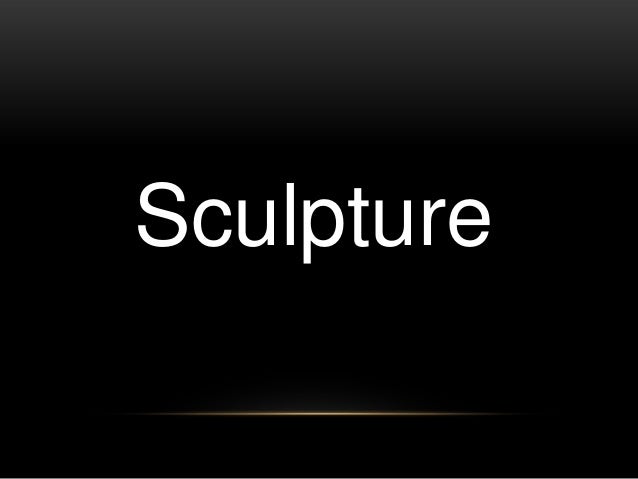The image is predominantly text-based with a simple design. At the center of the image is the word "Sculpture" in white uppercase letters, presented in a simple font with a capitalized "S." The black background varies slightly in shade, being lighter at the top and transitioning to a deeper black towards the bottom. Across the bottom of the image runs a goldish tan horizontal line, which brightens towards the center and fades towards the edges. No other objects or people are present in the image, giving it a minimalist appearance. The overall aesthetic suggests that it could be a title slide for a presentation, with its clean layout and limited color palette of white, golden brown, and black.